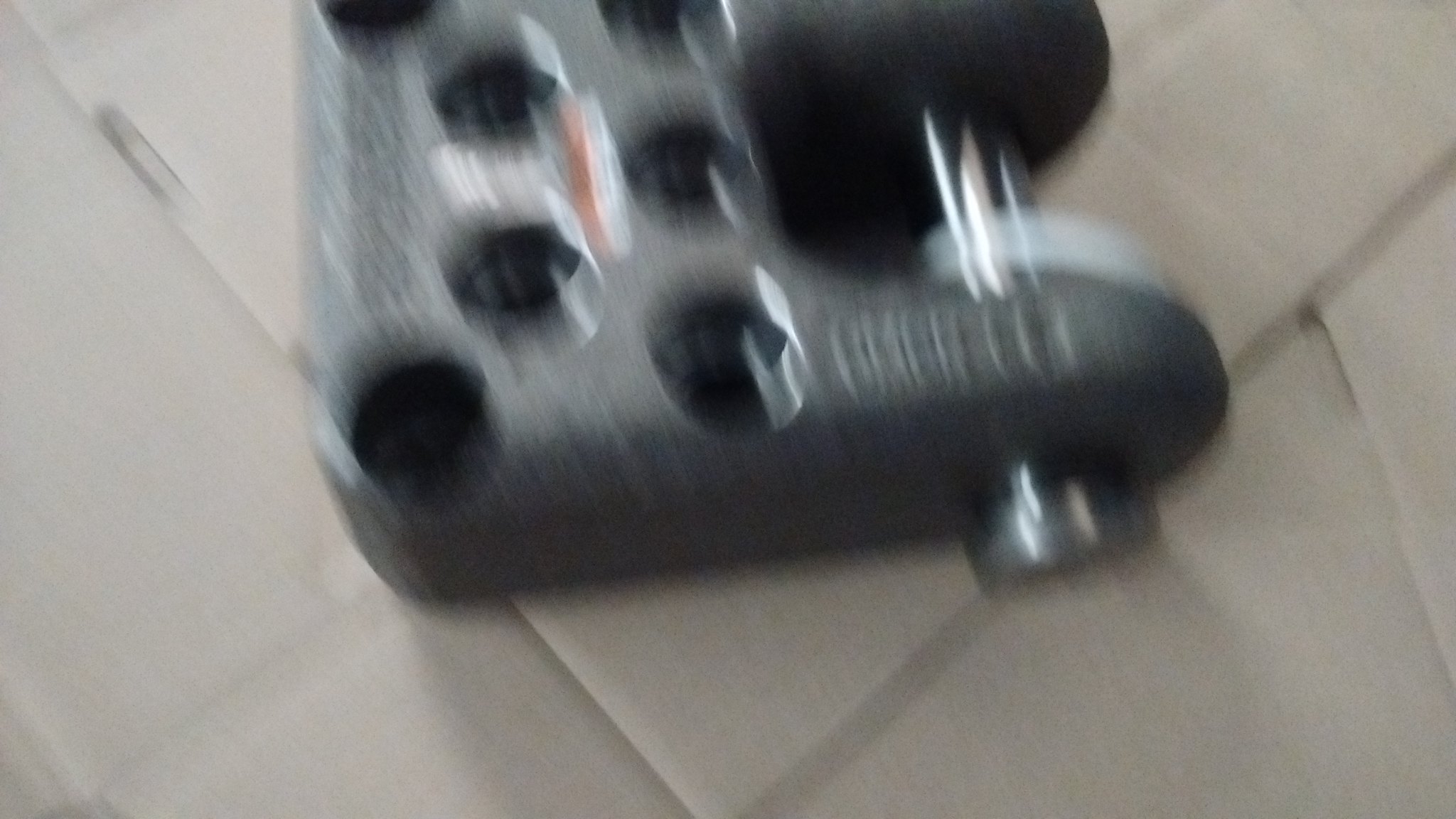A blurry photograph captures a mysterious black steel object in motion, possibly either falling or sliding across a white tiled floor accented with white or gray grout. The object, a solid piece of metal, appears hefty and is characterized by having seven distinct holes. While the exact nature of the object is unclear, it seems to be a part of a larger tool or machinery. There is some text faintly visible on the metal, but it remains illegible due to the blurriness. The overall scene conveys a sense of dynamic movement against a stark, tiled background.